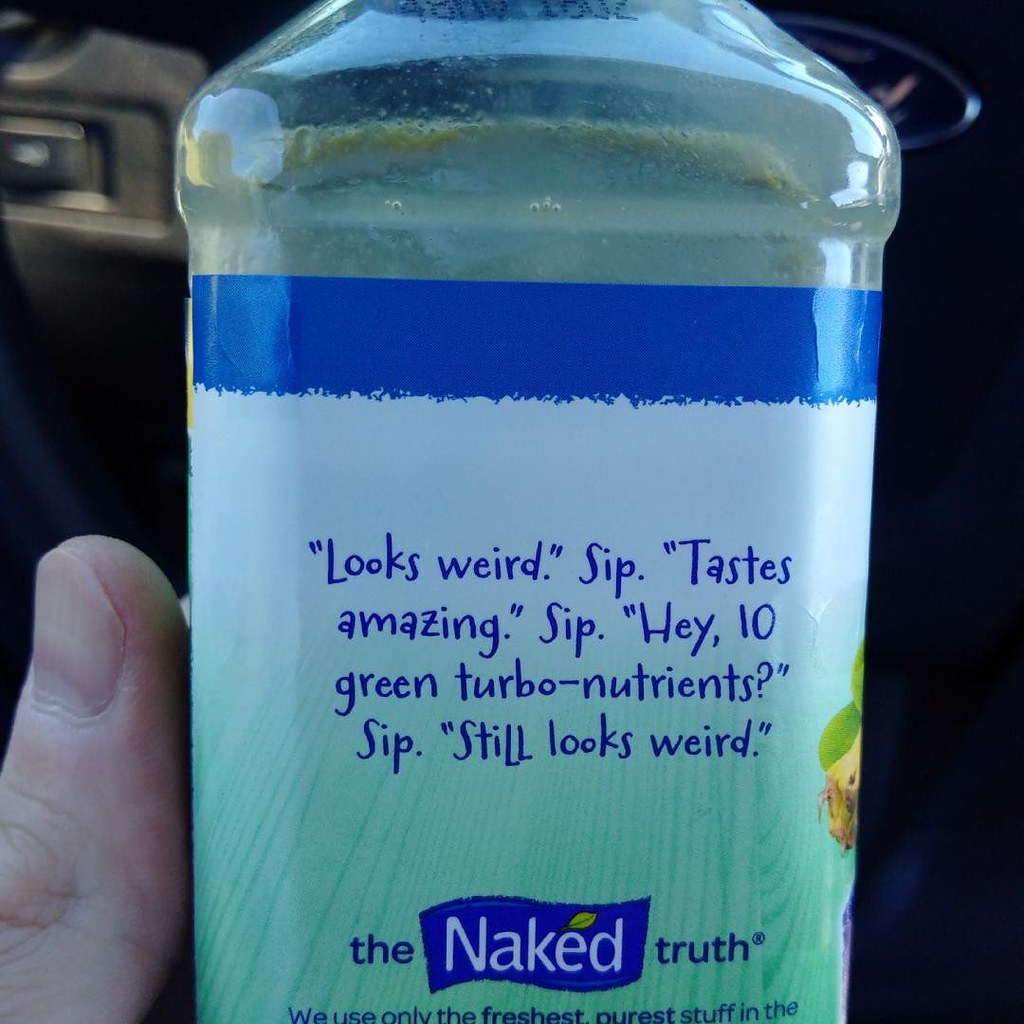This is a vivid color photograph featuring a label on a clear, opaque bottle. The label showcases an intricate design with a dark blue border at the top, characterized by a rough, jagged inner edge. The label smoothly transitions from a white background into a mint green shade, interspersed with diagonal, darker green lines, adding a dynamic texture. At the base of the label, elegant text reads, "The Naked Truth." Dominating the center of the label is a playful, handwritten-style font in dark blue, delivering a quirky narrative: "Looks weird. Sip. Tastes amazing. Sip. Hey, 10 green turbonutrients? Sip. Still looks weird."